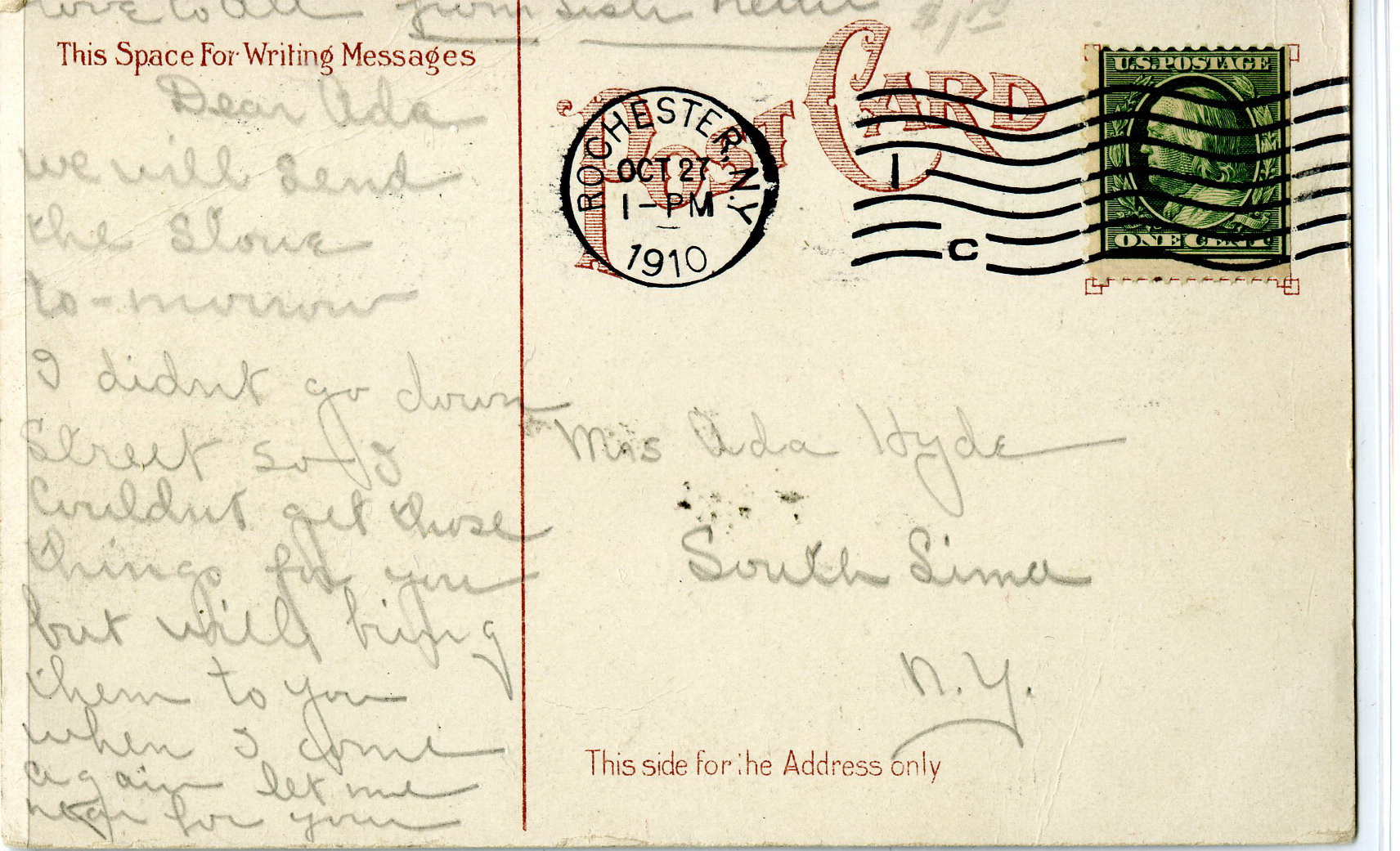This is a detailed photograph of the back of a very old, white postcard, postmarked in Rochester, New York on October 27th, 1910 at 1 PM. The postcard features a weathered appearance and a notable green one-cent stamp depicting Benjamin Franklin. At the top, the stamp is labeled "U.S. postage," with "one cent" inscribed at the bottom. The words "Postcard" appear in red ink, along with the postmark reading "Rochester, New York, October 27th, 1 PM, 1910."

Addressed to Mrs. Ada Hyde of South Sema, New York, the card bears the classic notation "This side for address only" on the right-hand side and "This Space for Writing Messages" in red on the left. The message, written in cursive pencil, reads, "Dear Ada, We will send the stove tomorrow. I didn't go downstreet, so I couldn't get those things for you, but we'll bring them to you when I come again. Let me know." The handwriting is elegant yet challenging to decipher, indicative of its age. Additionally, the left side of the card contains a partially visible inscription in cursive, beginning with "Love to All from," seemingly signed by "Sister," though the full text is cut off at the top.